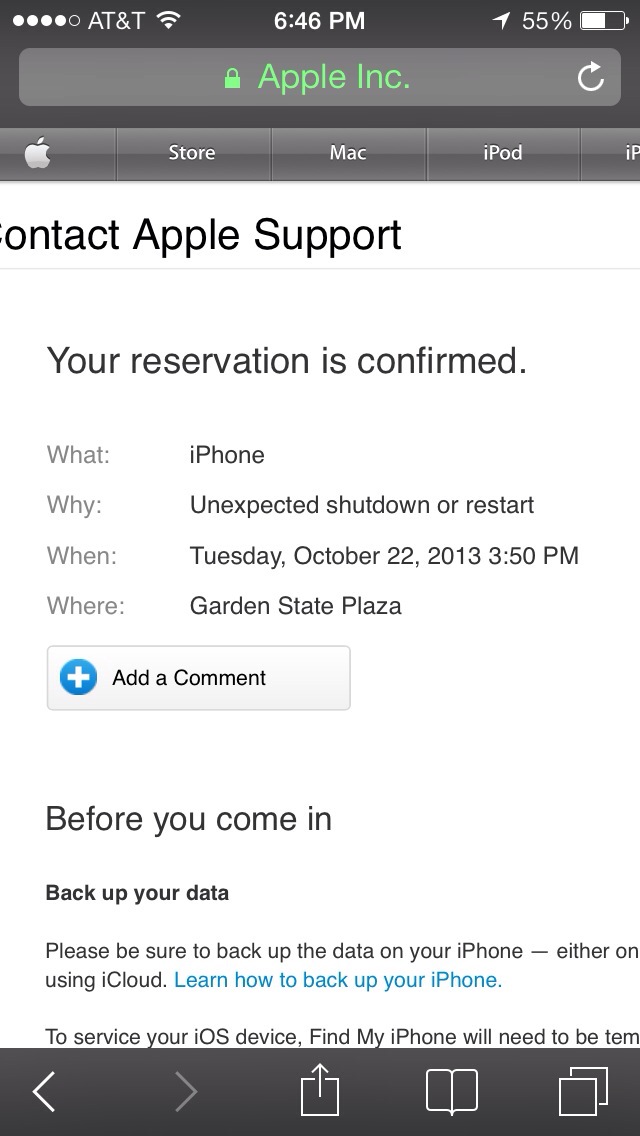This image is a screenshot of an Apple support reservation confirmation page viewed on an iPhone. At the top, the screen shows the carrier as AT&T, the time as 6:46 PM, and the battery level at 55%. Below, a green lock icon is followed by "Apple Inc.," and underneath, a navigation header with "Store, Mac, iPad, iPod." The targeted section confirms a reservation with the details: "What: iPhone, Why: Unexpected shutdown or restart, When: Tuesday, October 22nd, 2013, 3:50 PM, Where: Garden State Plaza." There is an option to "add a comment" indicated by a blue circle with a white plus sign. Instructions for preparation include "Before you come in, back up your data. Please be sure to back up the data on your iPhone either using iCloud," with a hyperlink for "learn how to back up your iPhone." Some text regarding servicing the device mentions "find my iPhone," with the remaining text cut off. The bottom portion of the screen appears to include a gray area with icons, though the details are not fully visible.